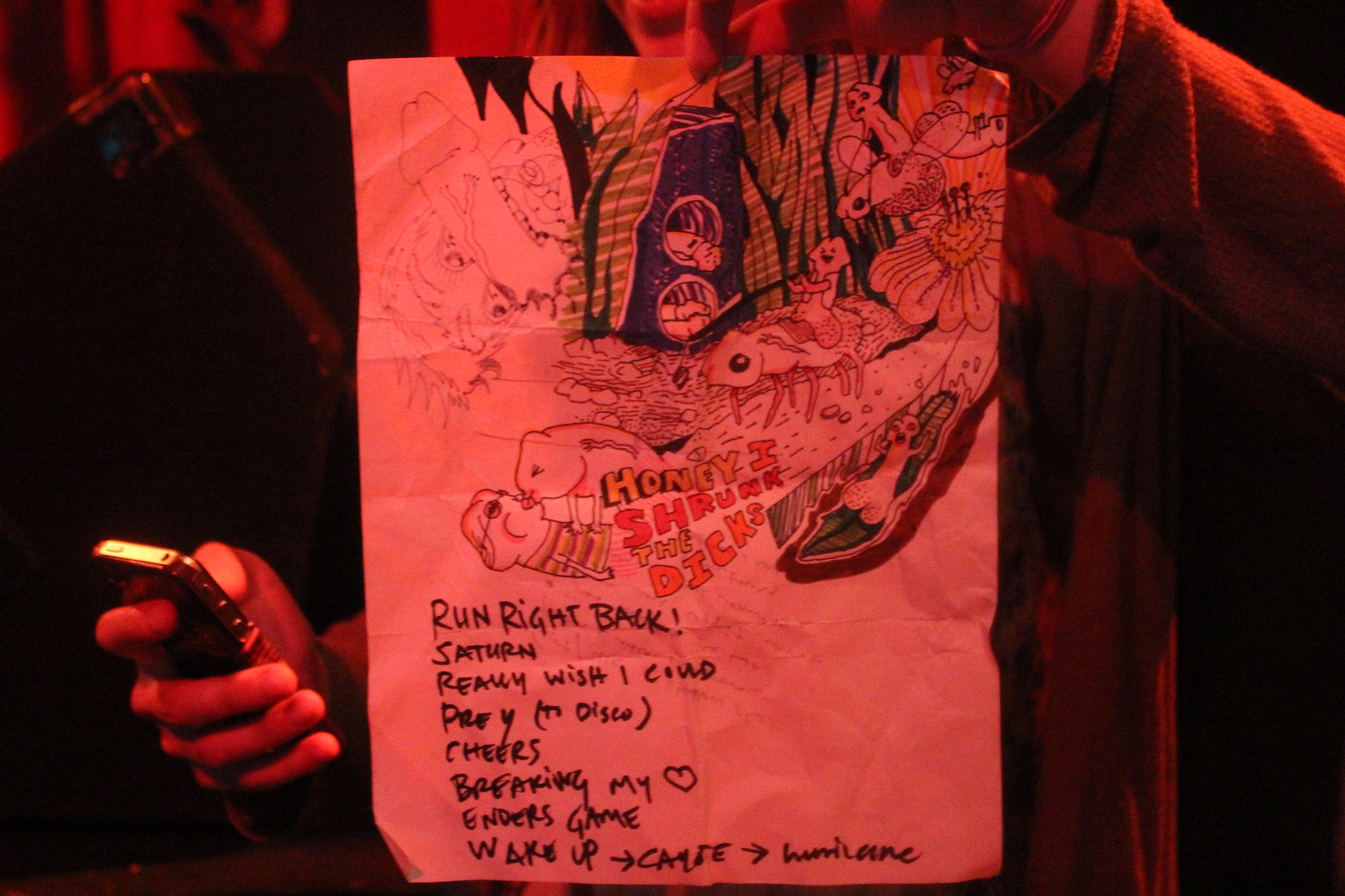The image portrays a man in a red-lit room, creating a landscape view with a reddish-black hue. At the center is a drawing featuring various animals, bugs, people, and penises in different states, contributing to its gross and potentially humorous nature. The drawing contains text at the bottom in black, with phrases including "run right back!", "Saturn really wish I could pray to disco," "cheers barfing my," a heart, "enders game," and "wake up for arrow," although some words are hard to decipher. The man holds up this bizarre and perhaps banned advertisement-like drawing with his left hand, while his right hand holds an iPhone, positioned in the lower left corner of the image. To the right of the drawing, the indistinct background somewhat reveals a torso and shoulder in the upper right corner, adding to the image's surreal atmosphere.